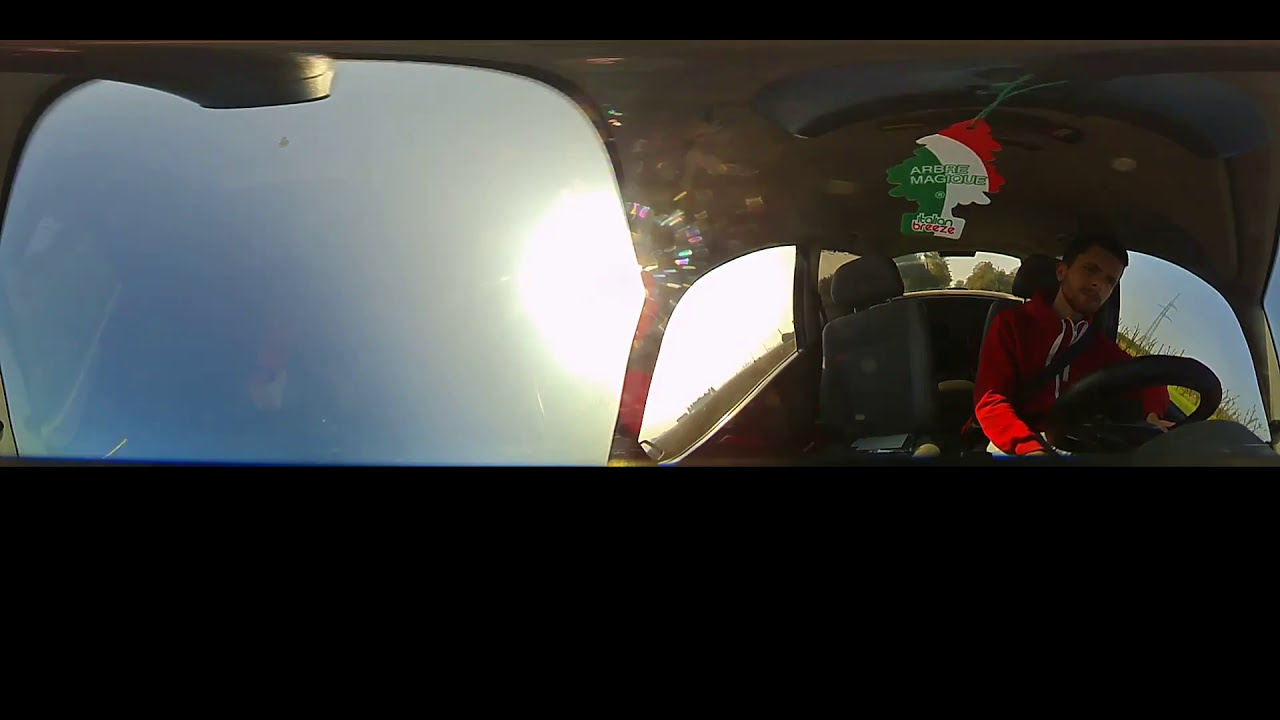In this image taken during the daytime, inside the vehicle, we see a scene through a slightly distorted windshield, likely due to the camera lens. The windshield shows a bright white sun with a faint yellow outline positioned at the center of the back. This sunlight casts reflections and highlights inside the car, illuminating various elements. Hanging from the rearview mirror is an air freshener decorated with red, white, and green stripes, and embossed with text that is unreadable except for parts starting and ending with the letters A and E, and another word starting with M-A-G and ending with E.

A man, wearing a red jacket adorned with white stripes down the middle, sits behind a black steering wheel on the right side of the image. He has short, trimmed black hair and appears to be gazing slightly downward. The passenger seat to his left is empty, featuring a smooth black leather texture. The ceiling of the car has an arched appearance. The vehicle's interior is complemented by vivid flashes of color—strips of yellow, fluorescent blue, and purple—originating from the sunlight and possibly reflective surfaces. The exterior scene beyond the car windows shows clear, sunlit skies, suggesting a bright and sunny day outdoors. The composition suggests a 360-degree perspective, allowing views of the back seats, various side windows, and parts of both the front and back of the car.